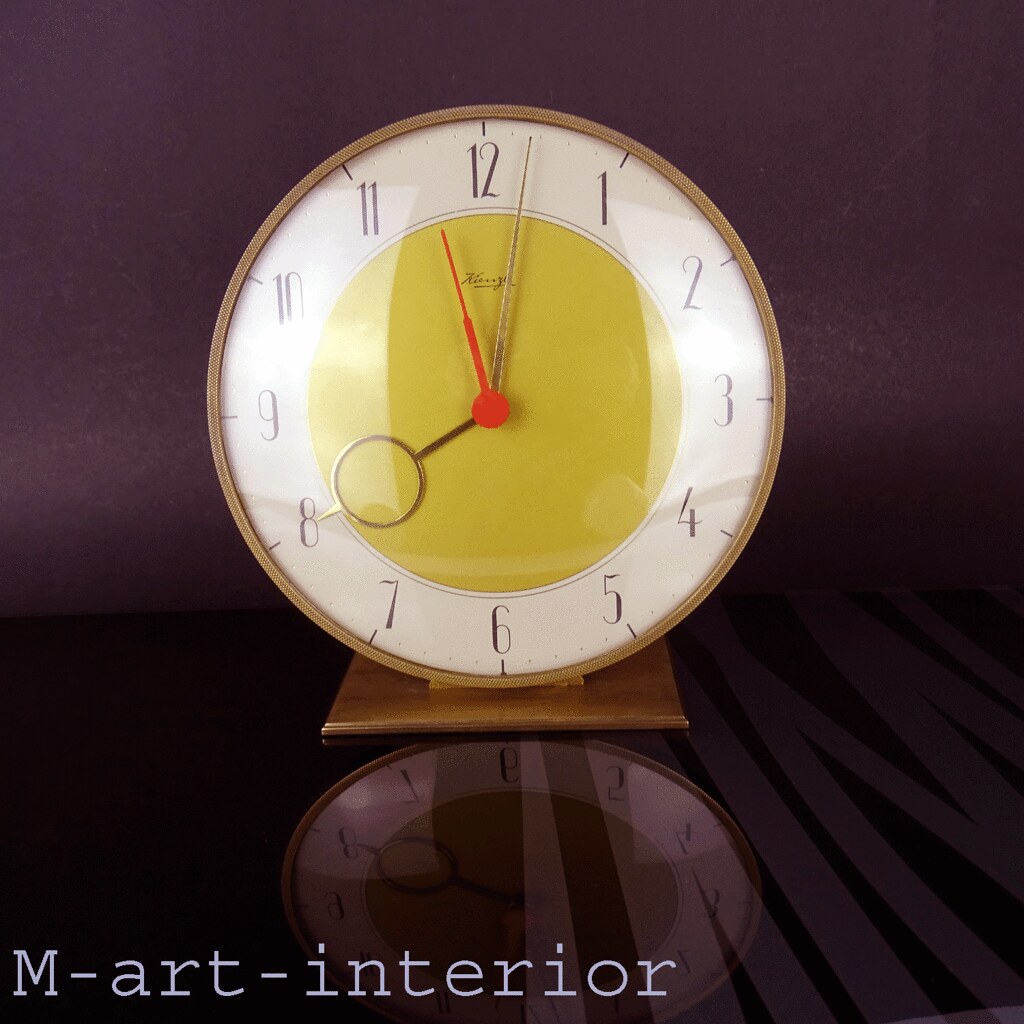The image features a small, bedside alarm clock with a distinctive design, set against a black and maroon background. The clock rests on a square, golden base that sits upon a reflective black surface, creating a mirrored effect below. The clock's exterior frame is wooden, matching the golden hue of the base. The circular face of the clock consists of concentric circles: an outer white circle with black numerical markings from 1 to 12, minute dots in between, and an inner greenish-gold circle. The brand name, written in cursive, appears but is too tiny to decipher. The gold hour hand has a distinctive circle, while the straight minute hand is also gold. A bright red seconds hand stands out sharply against the inner circle. The bottom left corner of the image displays the text "M-ART-INTERIOR."